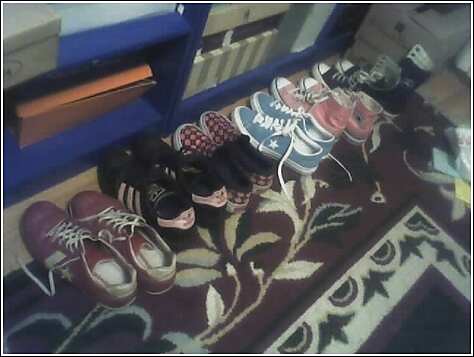The image showcases a domestic setting with a brown rug that has intricate floral patterns and a white inner border, adding to its detailed design. The rug spans diagonally from the bottom left to the top right, with various detailed floral motifs, vines, and leaves visible throughout. Sitting on this rug is an array of casual footwear, predominantly sneakers, arranged in a somewhat orderly fashion. Among the approximately seven pairs of shoes, there are notable brands and styles including Adidas, Vans, and multiple Converse shoes. Specific pairs include pink Chucks, burgundy and pink Vans, black Adidas with a colored rear, blue canvas shoes with white stars and laces, and some checked slip-ons. These shoes display a variety of colors like red, black, blue, and pink. In the top left-hand area of the photo, there is a blue bookshelf containing various boxes – likely shoe or cardboard boxes – adding to the domestic, lived-in feel of the scene. The bookshelf, painted blue, runs along the edge where the rug meets the wooden floor, indicating this might be an entryway where residents leave their shoes. Despite the low resolution and slight blurriness of the photo, the detailed description of the setting and items gives a clear sense of the environment captured.